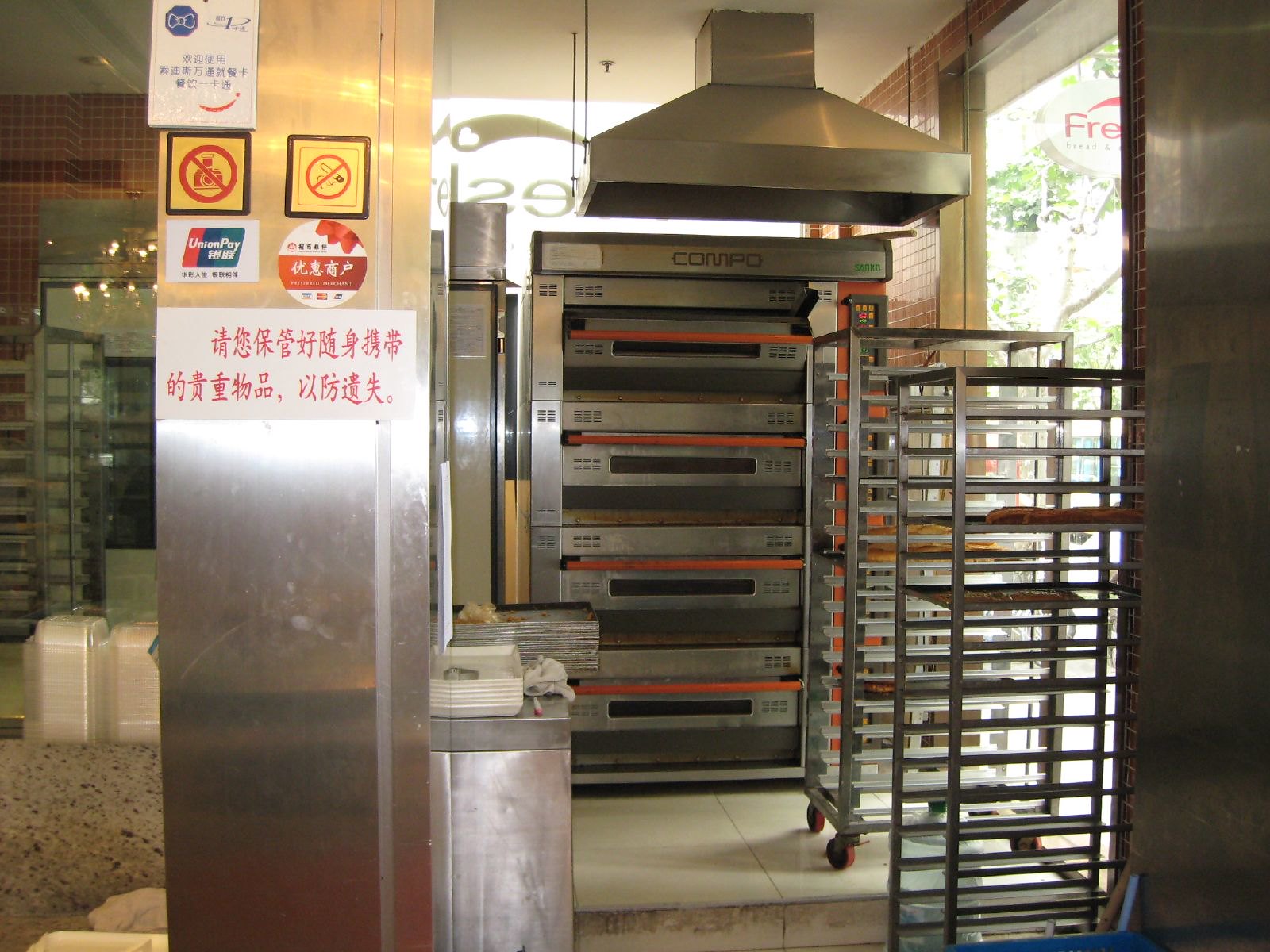The color photograph depicts the interior of a commercial kitchen or storeroom with an industrial feel. Central to the image is an industrial oven named "COMPO" with four opening doors, accents of orange lines, and a large extractor hood above, designed to vent heat from the area. To its right are tall, empty metal trolleys with multiple layers for trays. A wooden door is visible in this vicinity. To the left of the oven, a large post adorned with various stickers and signs featuring Chinese or Eastern writing stands prominent; these include yellow signs with red symbols and others in white that are unreadable. Additionally, there is a cabinet holding several stacked baking sheets, positioned next to metal racks and white containers. A blue bucket is placed in the foreground, and a red and white tiled wall can be seen towards the background, contributing to the industrial atmosphere.